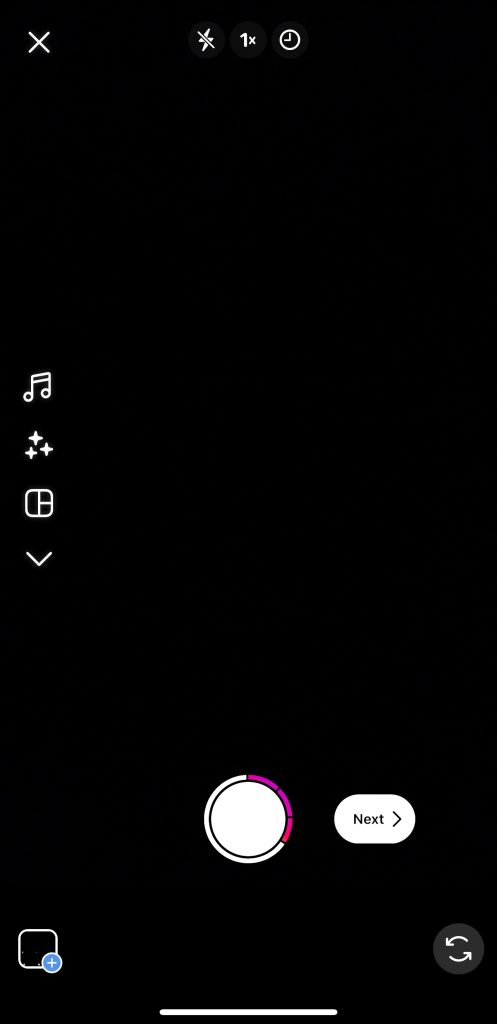The image appears to be a screenshot from a camera application interface on a smartphone. At the bottom center of the interface, a prominent white circular button is displayed, indicating the shutter button used to capture photos. At the top of the screen, there are a few icons commonly associated with camera settings. On the left, a lightning bolt icon, typically representing the flash function, is visible with a line through it, signifying that the flash is turned off. Next to the flash icon, the text "1x" is displayed, which likely refers to the current zoom level. Further to the right, there's an icon resembling a clock, potentially indicating a timer function. Adjacent to the main shutter button, on the right side, there's an oval-shaped button labeled "Max" in black text, possibly referring to a setting related to the camera's capabilities, such as maximum resolution or performance mode.